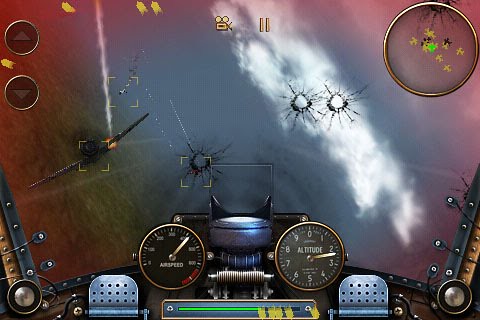The image is a detailed screenshot from a video game, providing a first-person view from inside an aircraft cockpit. Central to the scene are two gold-encased dials positioned directly in front of the player's viewpoint, indicating 'airspeed' on the left and 'altitude' on the right. Flanking these dials, on both sides of the cockpit, are what appear to be pedals. Above the instrumentation is the aircraft's windscreen, prominently displaying three bullet-hole-like openings, hinting at previous aerial engagements. On the left side of the image, an approaching aircraft is visible with a distinct yellow square marking. In the top left corner, up and down arrows are displayed, possibly indicating controls or status information. To the right, a circle contains various yellow and black plain-colored drawings or symbols, possibly representing mission objectives or alerts.